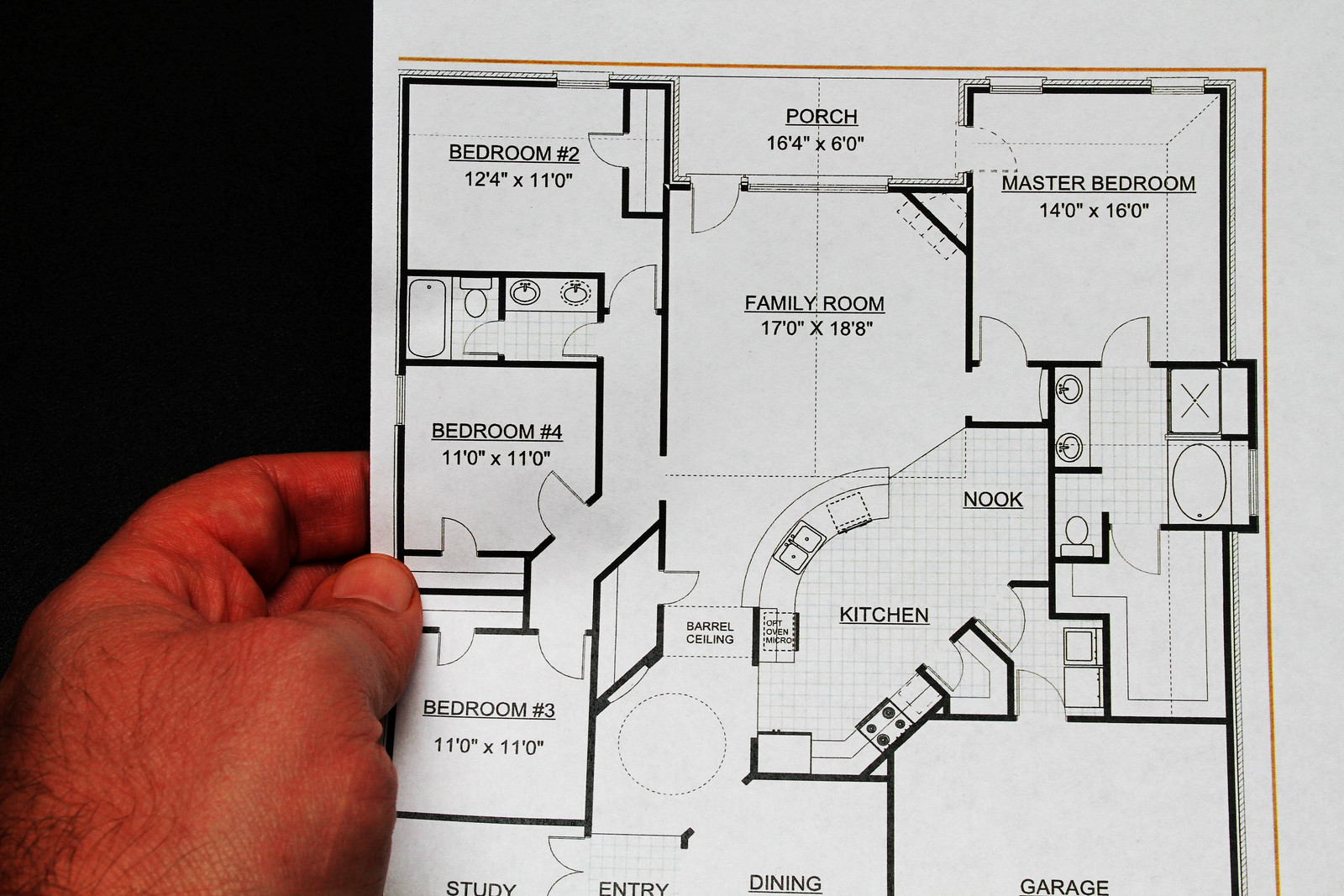In this detailed image, a person's left hand is seen holding a printed floor plan along its edge. The blueprint unfolds a comprehensive layout of a residential space. At the top, "Bedroom 2" is marked, adjacent to a porch area linked with the master bedroom. Central to the layout is the expansive family room. To the left of the family room, a hallway leads to Bedroom 2 and further down to Bedroom 4, which shares a wall with a bathroom. Continuing through the hallway, Bedroom 3 is positioned further down.

Towards the bottom of the floor plan, the spaces for a study, an entryway, and a dining area are clearly labeled. Near the family room, which connects to the kitchen, there is a designated nook area. Important details include the expansive master bedroom featuring a sizable bathroom equipped with dual sinks, a bathtub, and a shower.

In the bottom right corner of the plan, the garage is clearly marked. The floor plan also illustrates various door placements throughout the house, indicating the directional swing of each door for proper accessibility.